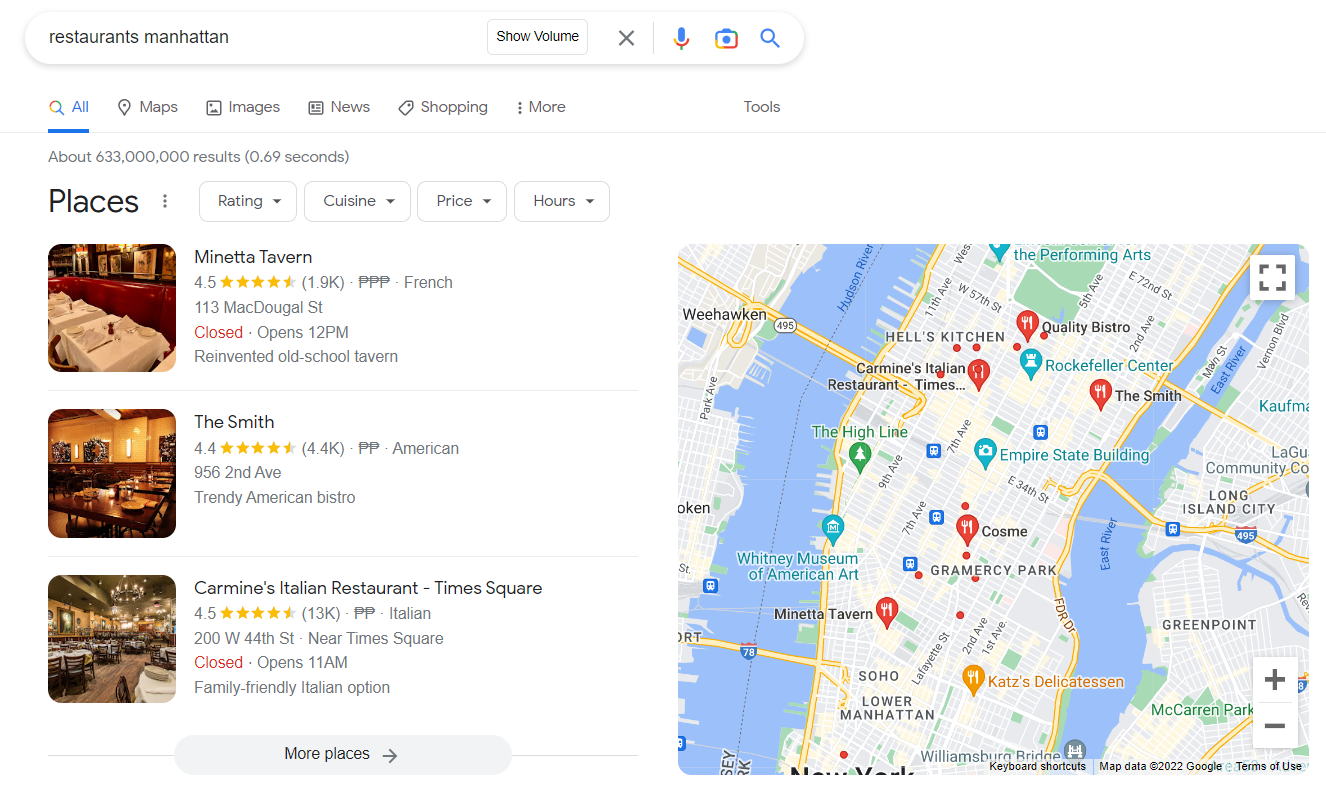The image displays a search engine results page for "restaurant Manhattan." On the right side, a detailed map with multiple drop pins highlights various restaurant locations. The left side showcases a list of restaurant options, with a search bar at the top left featuring the typed query "restaurant Manhattan." Next to the search bar, icons for "Show Volume," an "X" button, a microphone, and a search icon are present. Beneath these are tabs for "All," "Maps," "Images," "News," "Shopping," and "More," with the "All" tab underlined, indicating it is currently selected. 

Below, under “Places,” there are three featured restaurants accompanied by images and details. 

1. **Manita Tavern**: The first image displays dining tables adorned with white tablecloths. The restaurant has a rating of 4.5 stars and is noted to be "reinvented old-school tavern." It is currently closed and will open at 12 p.m.
   
2. **The Smith**: The second image shows a long dining table, seemingly lit by candlelight. It has a rating of 4.4 stars and is described as a "trendy American bistro."
   
3. **Carmine's Italian Restaurant**: The final image features a large dining room filled with tables, all draped in white tablecloths. The restaurant boasts a 4.5-star rating and is described as a "family-friendly Italian option." It is currently closed and will open at 11 a.m.

To the right of these listings are four dropdown menus labeled "Rating," "Cuisine," "Price," and "Hours" for further filtering the search results.